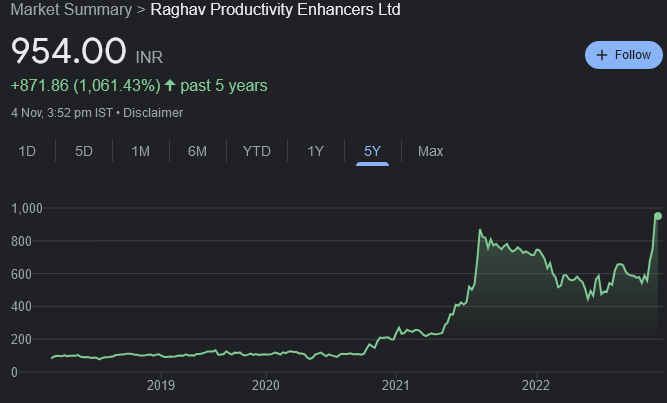### Detailed Description Caption

The image is a detailed snapshot of a stock market summary webpage, highlighting the performance of a company named Rag Cobb Protected Productivity Enhancers LTD. The market summary section, labeled in gray, prominently features the company's stock information.

At the top, an arrow points to the company's name, "Rag Cobb Protected Productivity Enhancers LTD," displayed in white text. Directly beneath this, the current stock price is shown as "₹954 INR" in green text, indicating a significant increase. An adjacent note records an impressive gain of "+871.86" in green, with the percentage change listed in parentheses as "(1000.061.43%)." An upward arrow indicates this performance is based on the past five years' data.

To the right of this section is a notable blue "Follow" button, allowing users to track the stock's performance actively. Below the stock price information is a timestamp in green, reading "November 4th, 3:52 PM IST," followed by a disclaimer in gray.

Further down the webpage, there are various visualization options for the stock's performance over different time frames—one day, five days, one month, six months, year-to-date, one year, five years, and maximum time frame—each represented by clickable tabs.

The stock performance graph below these tabs illustrates typical stock price movements with lines labeled for 1,800, 600, 400, and 200 units. A green line tracks the upward trend of the stock price over time, providing a visual representation of its growth. Along the x-axis, dates from 2019 to 2022 are marked, showing the timeline of the stock’s performance.

The color scheme of the webpage is predominantly black, green, white, and blue, providing a clean and professional look suitable for financial data presentation.